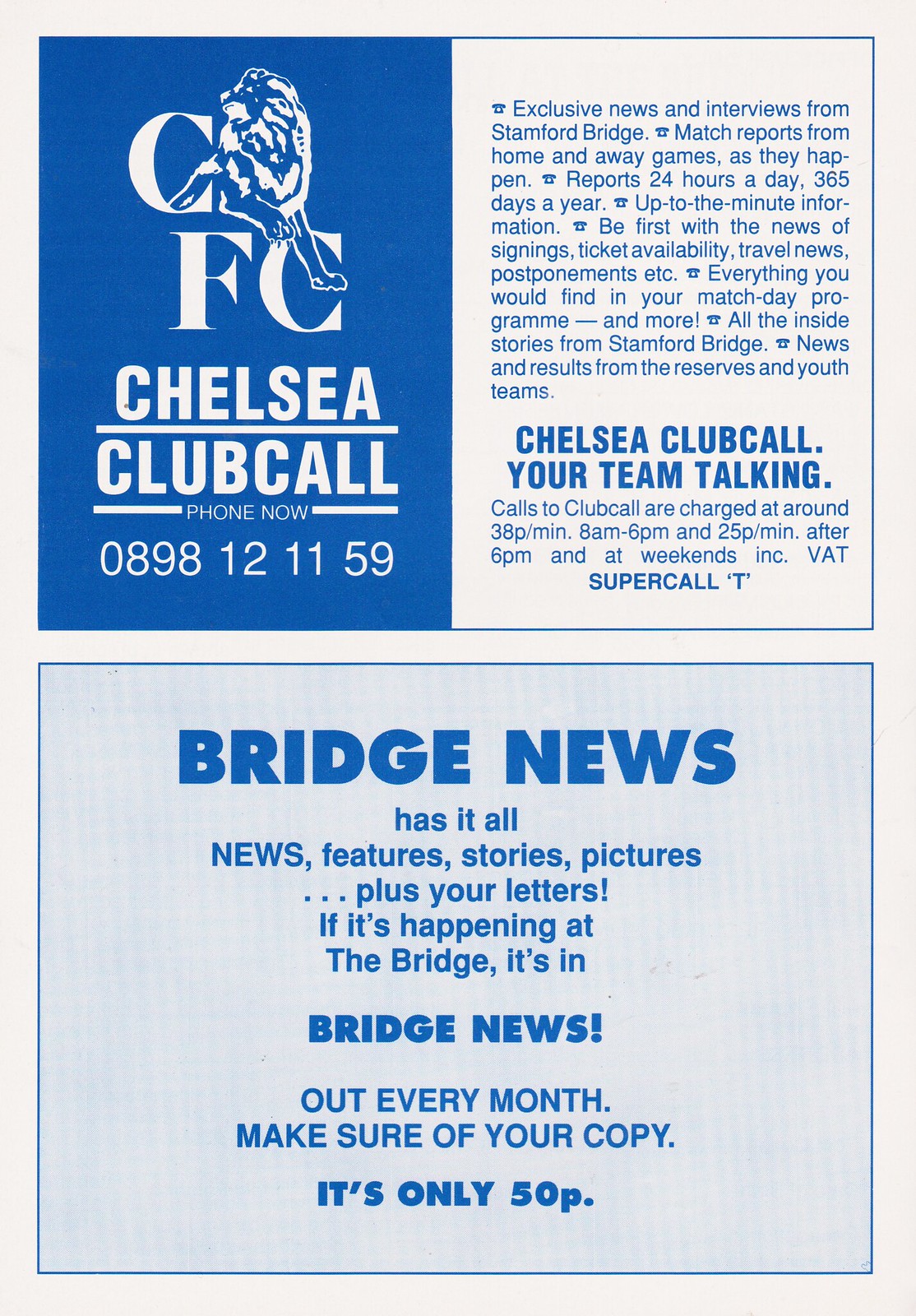The image features a vintage, newsletter-style pamphlet with a predominantly blue and white color scheme. The background is primarily white, with sections of deep blue. The top left section contains white writing that reads "Chelsea Club Call" followed by "Phone Now" and the phone number "0898-121159." Above these words, there's an animated picture of a lion that incorporates the letters "CFC." 

On the right side of the top half, the section promotes "Exclusive news and interviews from Stamford Bridge," along with match reports from home and away games, available 24 hours a day, 365 days a year. Beneath this, there are blue words on a light blue background, stating "Chelsea Club Call: Your Team Talking," followed by additional information.

The bottom half of the page displays a section labeled "Bridge News," which claims to feature news, exclusive stories, pictures, and reader letters. The text emphasizes that "if it's happening at the Bridge, it's in Bridge News" and highlights that the newsletter is released monthly and costs 50p. Blue borders frame the three distinct sections of content on the page. Additionally, there is a mention of call charges for using the club call, specified at 38p per minute from 8 a.m. to 6 p.m., and 25p per minute after 6 p.m. and during weekends.